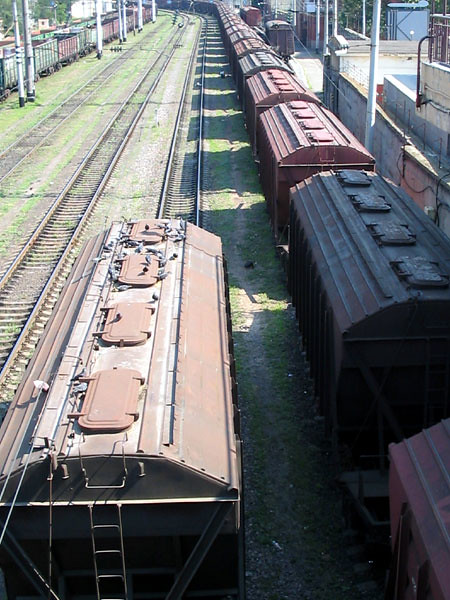The image depicts an expansive rail yard, viewed from above. In the upper right section of the photo, a wall runs parallel to the tracks. Tall electricity poles line the right edge, alongside a series of four railroad tracks that dominate the foreground. On the track farthest to the right, a continuous line of railroad boxcars, in hues of brick red, black, and muted gray, stretches into the distance. Each boxcar features four doors mounted on top, likely for loading from above. The second track from the right holds a single lone car, in contrast to the empty third track. To the left, two more tracks lie empty, while in the far-left background, more boxcars, some pink and green, are lined up, some appearing to carry coal or another dark material. Patches of green grass and brown dirt are interspersed between the tracks, adding a natural texture to the industrial scene. The boxcar in the foreground prominently displays a ladder fixed to its back, suggesting ease of access for maintenance or loading. This intricate view captures the varied elements and busy ambience of an active rail yard.